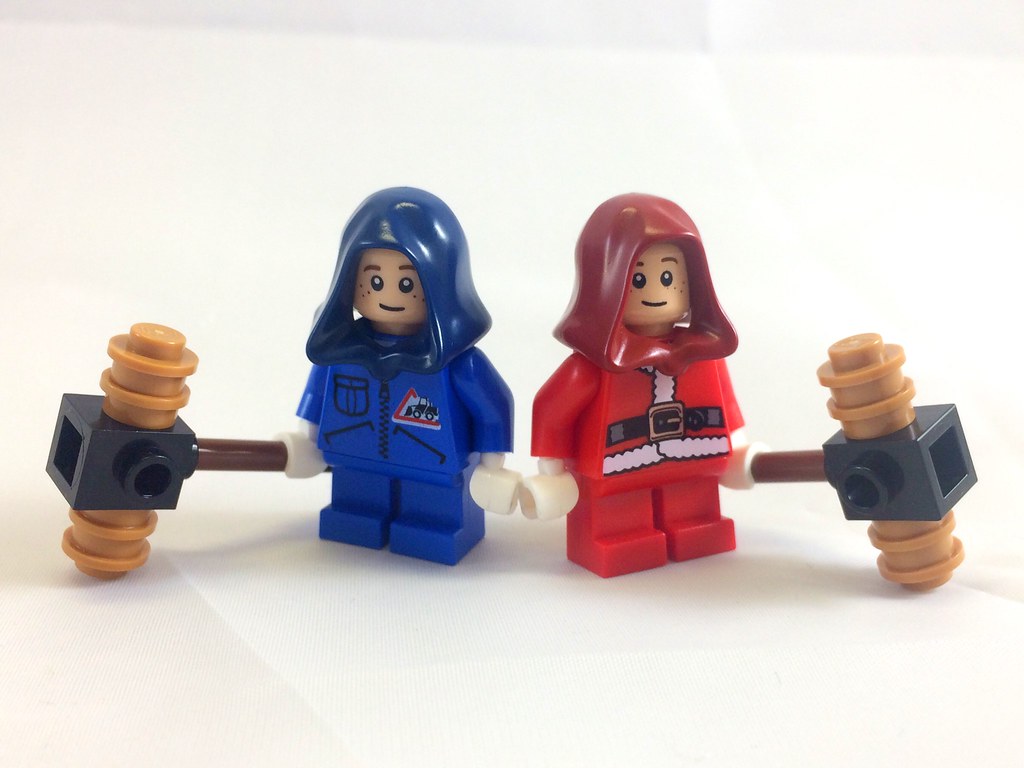In this horizontal photograph, set against a clean white background, two Lego figures stand prominently in the center. The figure on the left is dressed in blue, featuring a mechanics-style suit complete with a zipper down the front and a small emblem of a tractor encased within a white triangle outlined in red. This blue figure holds a distinctive hammer-like gavel with a brown handle and a black square middle, flanked by brown sections at the top and bottom. The figure on the right, clad in a classic Santa Claus outfit with white fur trim, a black belt with a gold buckle, mirrors the posture of its counterpart, also grasping an identical gavel. The characters, slightly angled away from each other, give the impression of facing opposite directions, while their hood-like hair completes the whimsical composition.